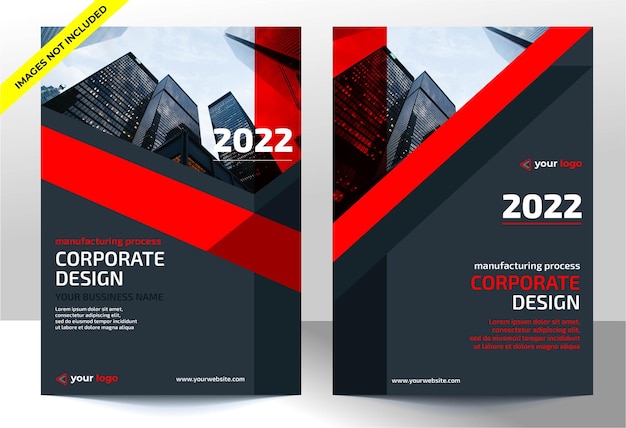This image showcases a horizontal mock-up of a corporate brochure's front and back covers, designed primarily in shades of charcoal gray, black, and vibrant red. Each side-by-side version highlights the potential layout for the company's promotional material. 

On the front cover, a dramatic photograph captures gray and black skyscrapers from a ground-up perspective, instilling an imposing sense of height. A bold red diagonal band divides the upper photograph from a charcoal gray block beneath, which contains a text area in white and black and reserves the lower left corner for a company logo. Additionally, a band along the right edge transitions from red at the top to deep charcoal at the bottom, seamlessly blending into the design.

The back cover mirrors this aesthetic with slight variations. An analogous cityscape photo, sans two buildings from the original, maintains the theme. Above the year "2022" and the text "Manufacturing Process, Corporate Design," set in red and white, the design incorporates areas for additional copy. The yellow angled banner at the top right corner that reads "Images Not Included" appears on both covers, echoing a professional disclaimer.

Together, these prototypes illustrate a sleek, modern brochure layout that emphasizes visual appeal and corporate branding.